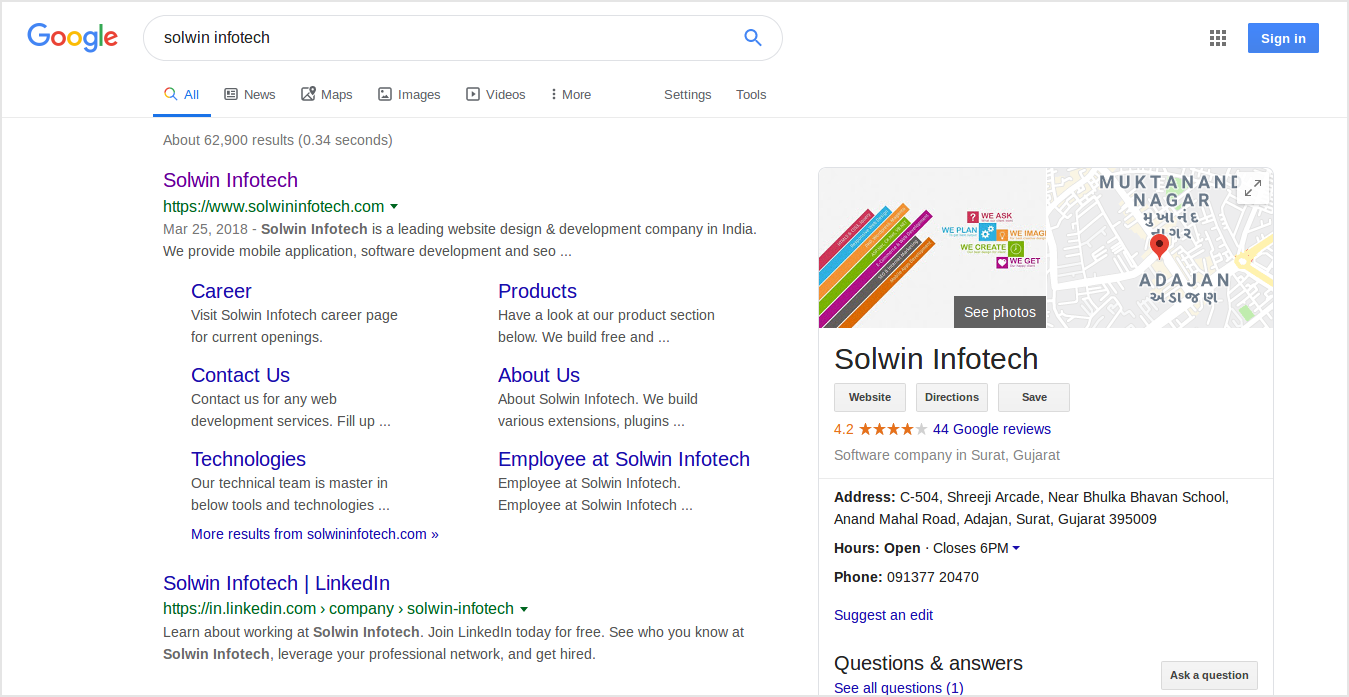The image displays a Google search results page. At the top left, there is a Google icon. The search bar contains the query "Solent Infotech." Just below the search bar, it indicates that there are approximately 62,900 results found in 0.34 seconds.

The first search result is prominently highlighted. The title, "Solent Infotech," appears in purple, and below it, the URL "https://www.solentinfotech.com" is displayed in green. The snippet of information provided under the URL reads, "March 25th, 2018, Solent Infotech is a leading website design and development company in India. We provide mobile applications, software development, and..."

Following this, there are several blue links with corresponding black descriptions:
- "Career" in blue, followed by "Visit Solent Infotech career page for current opening."
- "Contact Us" in blue, followed by "Contact us for any web development services."
- "Technologies" in blue, followed by "Our technical team is master in below tools and technology."

The overall design highlights the comprehensive range of services provided by Solent Infotech, including website design, mobile applications, and software development, emphasizing their expertise and available career opportunities.